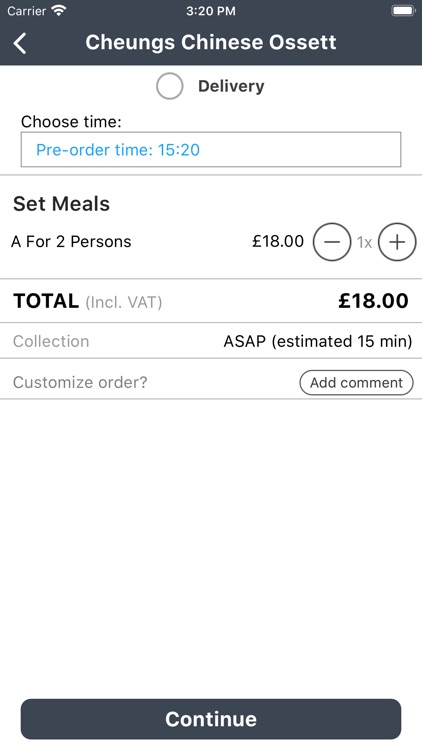This is a detailed screenshot of the "Cheung's Chinese Asset" website. At the top, the header is dark grey with the text "Cheung's Chinese Asset" prominently displayed in white. The webpage features a clean design with a white background. Immediately below the business name, there's a "Delivery" bubble indicating the service available. Following this, there's an option to "Choose Time" with a text bar displaying "Pre-order time 15:20" in blue.

The next section showcases a set meal for two persons, priced at £18. This meal option can be customized, and the price is clearly bolded, stating "£18 total". Additionally, there is an option for "Collection ASAP" with an estimated preparation time of 15 minutes, highlighted. 

Just below, there's an "Add a Comment" tag allowing for customization notes. There is noticeable spacing before reaching the bottom of the webpage, which features a grey "Continue" button with the text "Continue" in white, providing a clean call-to-action for users.